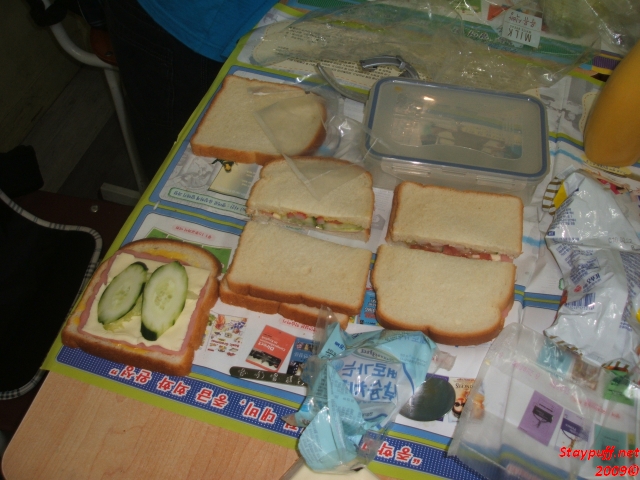The image depicts a detailed scene of someone preparing lunch at a wooden table. In the top right corner, a person's elbow is slightly visible, suggesting they are leaning on the table. The table is covered with a plastic mat or tablecloth that features Chinese characters and images, providing a colorful backdrop. A variety of breads and sandwiches are arranged on the table. One piece of bread is plain, another has cheese and two slices of cucumber, while several completed sandwiches are also visible, with some cut in half to reveal indistinct vegetables in red and green hues. There are various Tupperware containers—one with a blue-edged lid—and other indistinguishable items scattered around. The overall scene is vibrant, with an array of colors and elements indicating an active and diverse lunch preparation. In the very bottom right corner, partially obscured, the text "staypuff.net2009c" appears faintly in red.